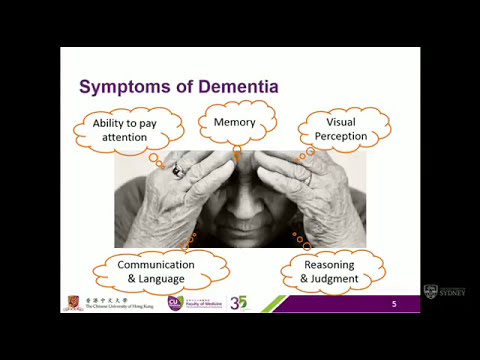The image is a detailed presentation slide illustrating the symptoms of dementia. The slide is bordered with a thick black frame roughly an inch wide and features the title "Symptoms of Dementia" in purple font at the top. Central to the slide is a poignant black-and-white photograph of an elderly person, identifiable by their wrinkled hands, with their head resting in their hands in a thoughtful pose. Surrounding this image are orange-edged thought bubbles containing the symptoms of dementia: "Ability to Pay Attention," "Memory," "Visual Perception," "Communication and Language," and "Reasoning and Judgment." The overall background of the slide is white, complemented by a decorative strip at the bottom right: a slanted purple section alongside a lime green segment, both marked with the numbers 35 and 5, respectively. Additionally, there are some small icons in the bottom left, accompanied by some writing, giving the slide a structured yet solemn presentation.